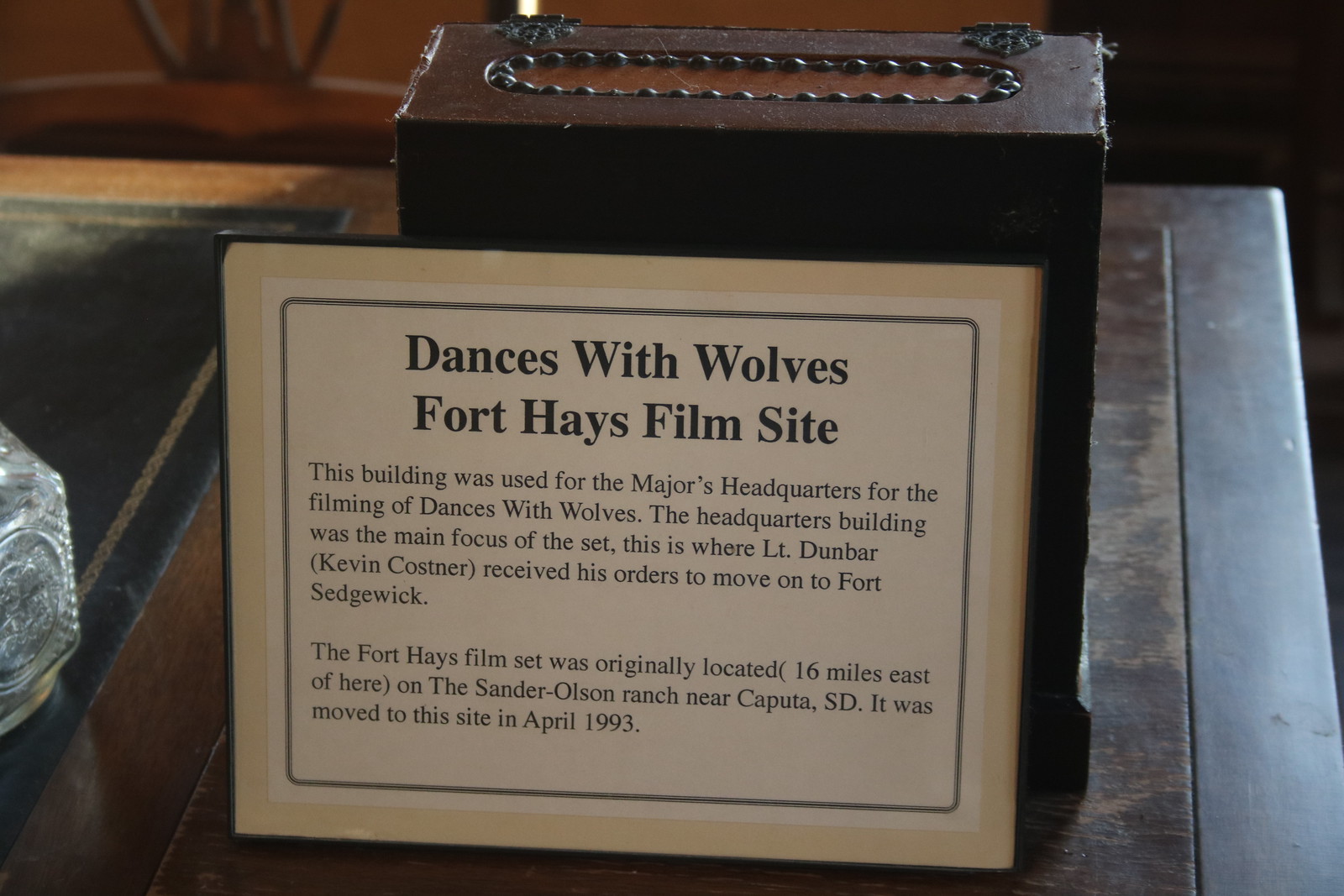The image showcases a sign placed on a brown wooden table, leaning against a brown leather box adorned with studs and featuring two latches on the top. The box, which has an opening at the top, sits prominently with the sign. The sign itself is framed and bordered, starting with a light black border, followed by cream, white, and then another black border. The text on the sign reads "Dances with Wolves, Fort Hayes Film Site." It provides detailed historical information, stating that the building featured was used as the Major's headquarters for the filming of "Dances with Wolves." This headquarters building was the central focus of the set where Lieutenant Dunbar (Kevin Costner) received his orders to move on to Fort Sedgwick. Originally, the Fort Hayes Film Set was located 16 miles east on the Sander Olsen Ranch near Caputa, South Dakota, before being relocated to this site in April 1993. The background includes additional wooden furniture and dark materials, accentuating the significance of the framed informational sheet in the image.